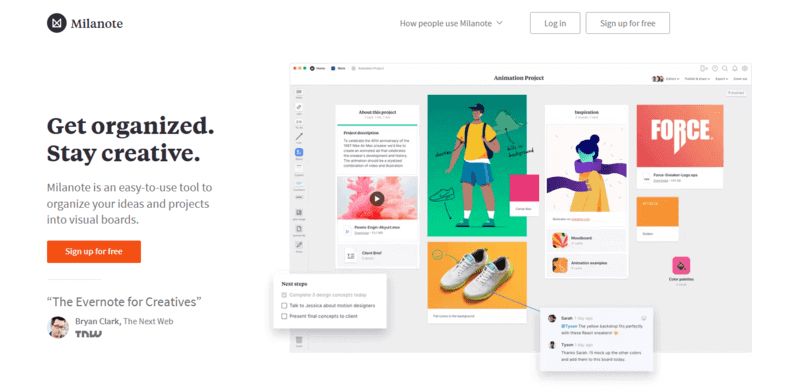At the top of the image, there's a black circle with an icon in the middle and the word "Mylanote." On the right side, text reads "How people use Mylanote." There are two buttons underneath: "Login" and "Sign Up for Free." Below, to the left, the text "Get organized, stay creative" is followed by a brief description: "Mylanote is an easy-to-use tool to organize your ideas and projects into virtual boards." An orange button below this text also says "Sign Up for Free." Further down, there's a review that reads, "The Evernote for creatives. — Brian Clark, The Next Web (TNW)." On the right side of the image, a web page is displayed with a couple of small, blurry pop-up boxes. The visible images include a pair of shoes and an illustration of a person wearing blue shorts, a gold shirt, a black baseball hat, and a book bag.